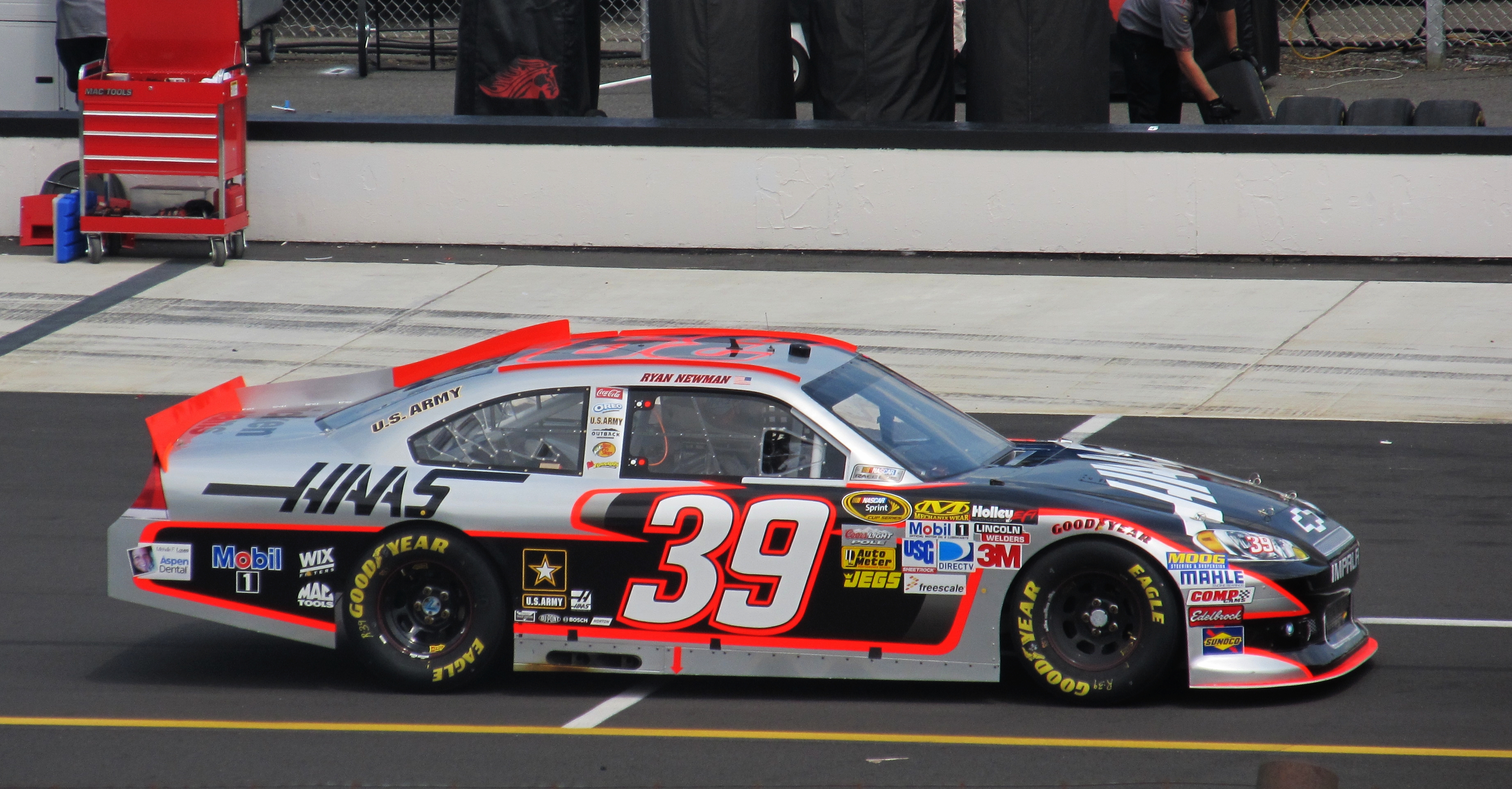This photograph captures a dynamic scene at a NASCAR race featuring Ryan Newman's stock car, numbered 39. The car, a striking blend of silver, black, and vivid orange, prominently displays a variety of sponsor logos, including Haas, U.S. Army, 3M, Mobil 1, and many others such as NASCAR, Spirit, Autometer, Jags, Freescale, DirecTV, USG, Holley, Lincoln Welders, Moog, Molly, Comp, Edelbrock, Sunoco, Oreo, Coca-Cola, Outback Steakhouse, and possibly Red Bull. Ryan Newman's name is seen on the vehicle, confirming his ownership of the car. It rides on black Goodyear tires adorned with the recognizable yellow Goodyear logo. The car is situated on the dark tarmac of the pit stop, bordered by a white barricade. In the background, there is a red toolbox on wheels and crew members handling tires, adding to the bustling atmosphere of the race event.